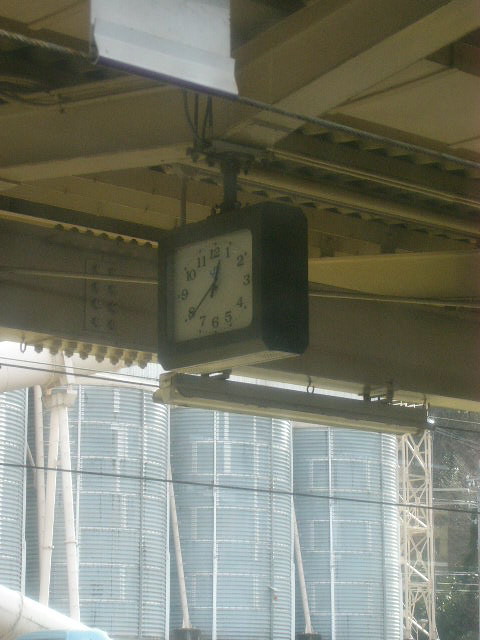This detailed photograph captures an industrial-style building with prominent tan-colored girders and beams crisscrossing the ceiling. Suspended from one of these beams is a black clock mounted on a cylindrical pole. The clock itself is encased in a substantial rectangular black frame, approximately an inch or two thick. Its white face features numerals in a standard numerical format from 1 to 12, with black hour and minute hands clearly visible. In the backdrop, a row of windows with open blinds provides a hint of the outside environment, including aluminum industrial silos supported by white structures. Below the clock, a fluorescent light fixture hangs prominently. Additionally, heavy steel beams with massive bolts are discernible, reinforcing the industrial atmosphere of the setting.